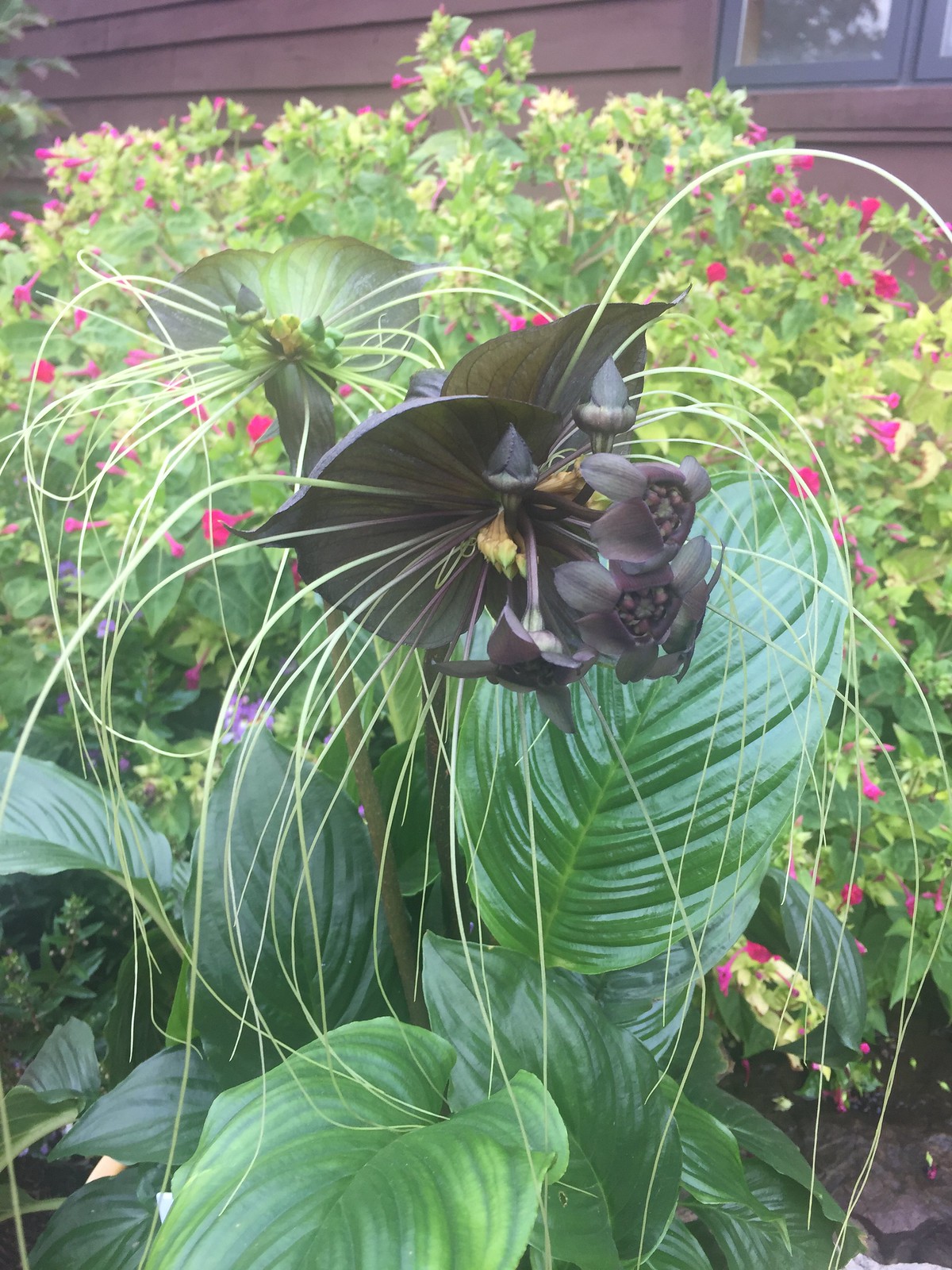The image, set in portrait orientation, showcases a striking and exotic garden scene. Central to the composition is a dark purple, almost black flower with large petals. From the base petals, smaller versions of the flower emerge, each exhibiting multiple petals and surrounded by long, light green tendrils extending outward. A secondary flower, slightly less bloomed, is positioned behind the main flower. Both flowers are supported by thick, sturdy stalks and framed by large, shiny, dark green leaves reminiscent of elephant ear plants. 

In the background, a lush bush filled with green leaves and reddish-pink flowers adds a vibrant contrast to the dark central flower. Further back, the brown wooden siding of a building provides a rustic backdrop. The window on the top right reflects the surrounding landscape, including glimpses of trees, the blue sky, and white clouds. The overall scene captures a beautifully detailed and harmonious blend of natural elements against a charming architectural setting.